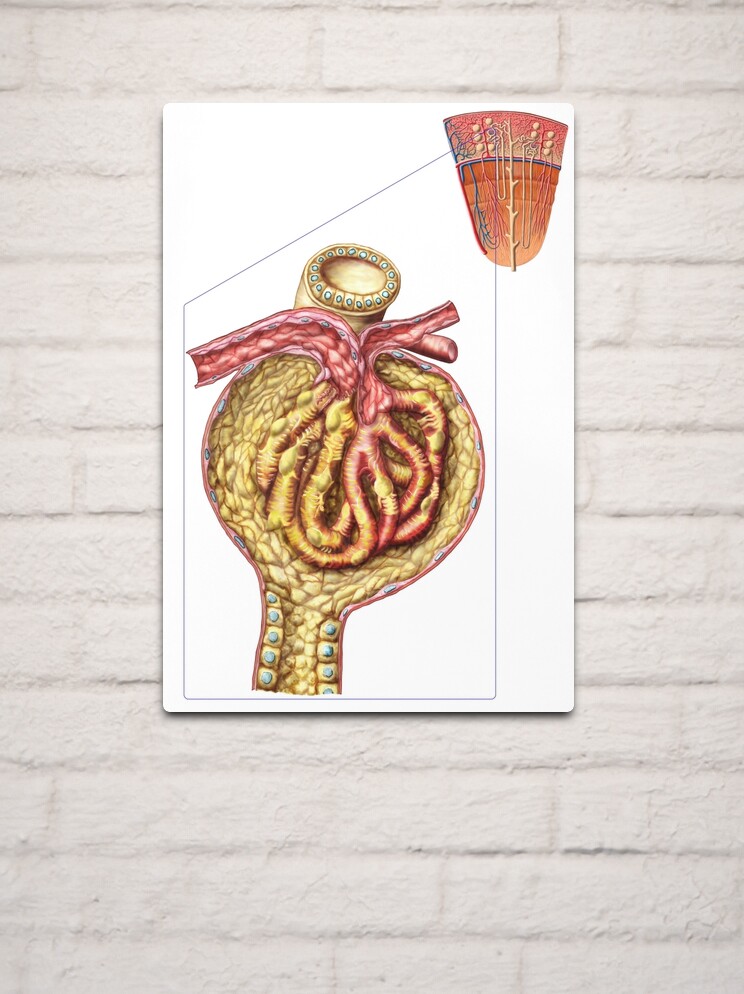This detailed illustration, possibly digital, is mounted on a white brick wall. The illustration itself is on a flat white surface positioned against the textured brick backdrop. The image appears to be an anatomical drawing, potentially depicting a zoomed-in section of the human body. The focal point of the illustration seems to feature a complex, tube-like structure resembling glandular or cellular tissue, possibly a sebaceous gland or part of the skin. The intricate details within the image suggest an internal composition, perhaps akin to a cell structure or an autopsy cutaway but without visible animal parts. There's a thin blue highlighted area near the top, emphasizing a specific segment of the anatomy. The entire depiction is devoid of any labels or text that would clarify its exact nature.